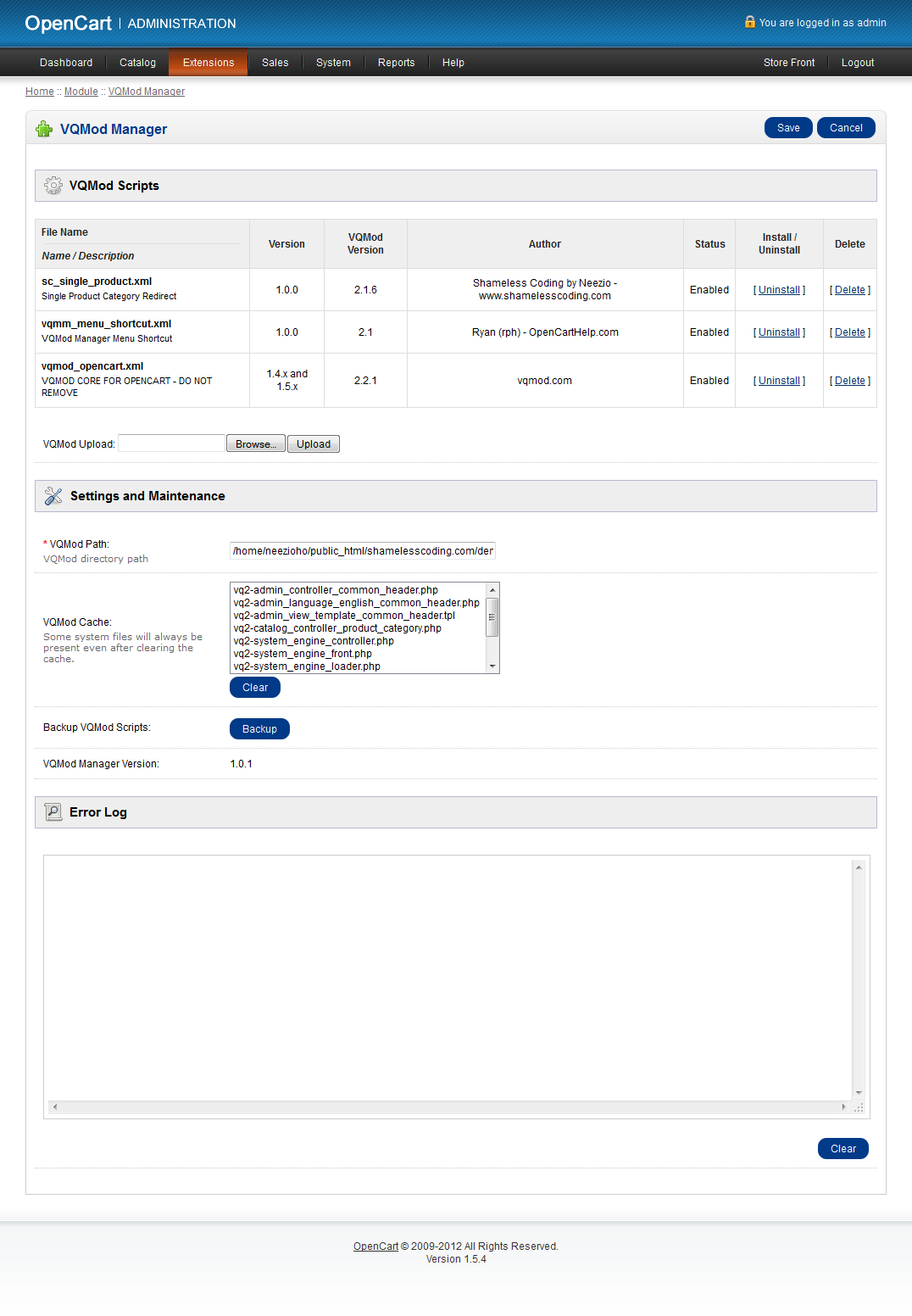Screenshot of the OpenCart Administration panel logged in as Admin, showcasing various sections including Dashboard, Catalog, Extensions, Sales, System, Reports, Help, and VQMod Manager. The VQMod Manager interface displays a grid with columns such as File Name, Name Description, Version, and Author. Examples include "Single Product" by "ShamelessCoding (Ryan Ripp)," compatible with OpenCart versions 1.4.x to 1.5.x, and version 2.2.1 by Nezio from ShamelessCoding.com. The admin interface lists multiple states for modules, including "Enabled," "Uninstalled," and options for "Delete." The menu also features VG Mod Upload options with "Browse" and "Upload," settings for maintenance tasks, and management of VQMod paths and captcha settings. The panel includes a version information section showing OpenCart version 1.5.4 and a helpful link to OpenCartHelp.com. The footer notes are from OpenCart, copyrighted from 2009-2012, indicating all rights reserved.